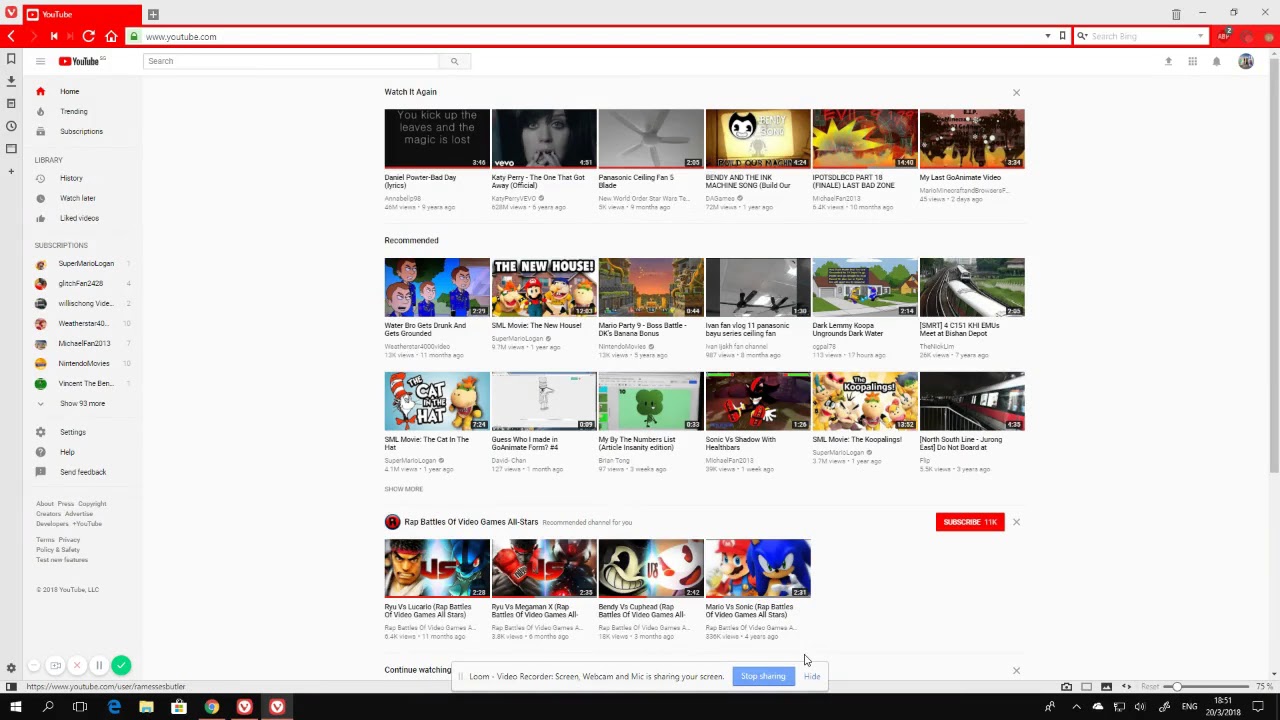This image is a detailed view of a YouTube homepage displayed in a browser window. In the upper-left corner of the window, there's a red square with a white letter "V" inside, suggesting it's likely a custom browser or extension icon. The browser's tab is accentuated by a red background, featuring a white YouTube play button icon, the text "YouTube," and a gray plus sign to its right. Typical browser control buttons for minimizing, restoring, and closing the window are present in the upper-right corner.

The address bar is white and prominently displays "www.youtube.com." To the right of this, there's a small section labeled "Search Bing," indicating that this is likely the Microsoft Bing browser. 

The YouTube homepage itself has a white background with a light gray column on the left side, where navigation options are available. These options include Home, Trending, Subscriptions, History, Watch Later, and Liked Videos. Underneath, there is a section titled "Subscriptions" displaying channels like Super Mario Logan and Ghost Fan 2428, among others.

The main content area of the YouTube page shows six videos in a single column under a "Watch It Again" section. Below this, there is a "Recommended" area laid out in two rows, totaling twelve videos. At the very bottom of the homepage, there is a section titled "Rap Battle: The Video Games All-Star" featuring four additional videos.